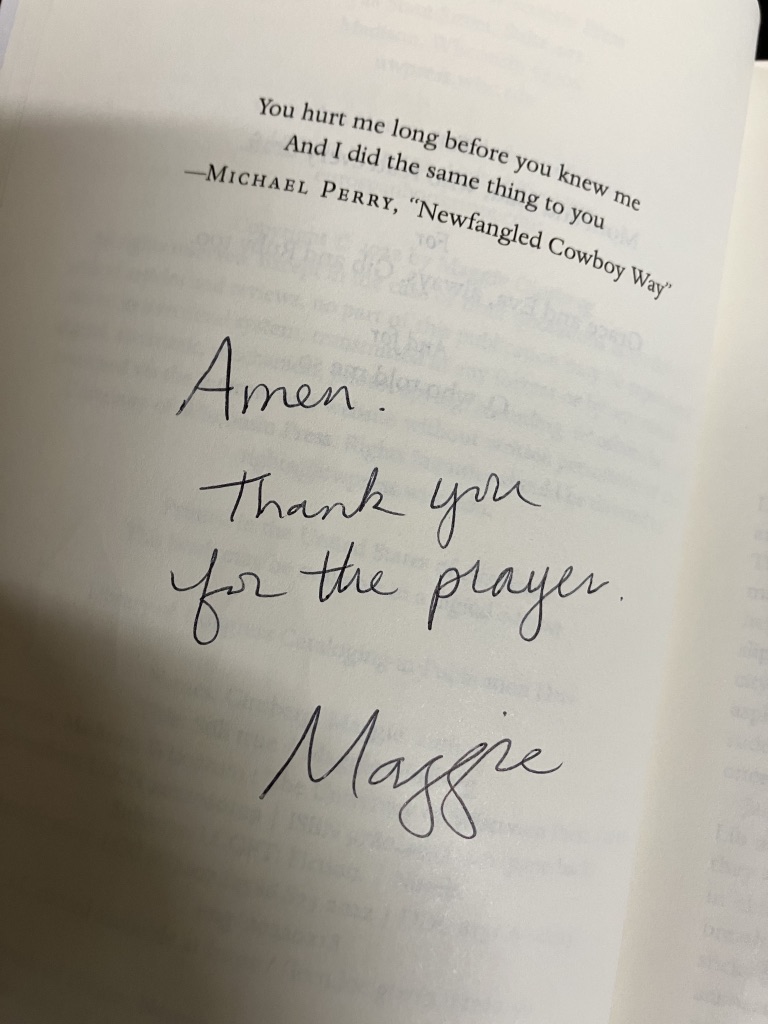The photo captures a white book page, possibly a dedication or the first page of a text. At the top of the page, a printed quote reads, "You hurt me long before you knew me, and I did the same thing to you." Below the quote, the author is identified in block capitals as MICHAEL PERRY, followed by the phrase "Newfangled Cowboy Way." Underneath this printed text, someone has handwritten in black pen, "Amen. Thank you for the prayer." and signed it as Maggie. The text appears very centered on the page, and due to the thinness of the paper, the print from the following page is faintly visible through it. The overall aesthetic is black and white, suggesting a thoughtful or sentimental context for the image.